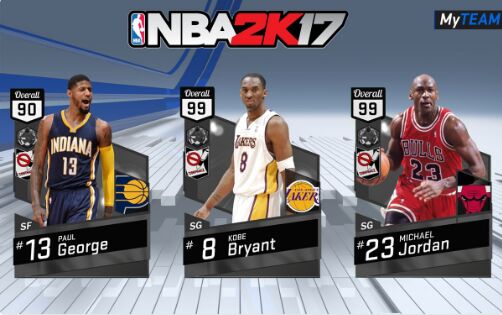The image features a vibrant NBA-themed layout. At the top, there is the iconic NBA logo followed by the text "NBA" in large print. Next to it, the title "2K" is prominently displayed in bold red letters, and "17" appears in sleek gray print. In the upper right corner, a black rectangle contains the word "MY" in white, followed by "TEAM" in all caps and blue.

Below this header, there are three basketball card-like images of different legendary players. 

- On the left, the first image features a player donning an Indiana Pacers jersey, with the number 13. He is looking to the right and an overall rating, albeit somewhat blurry, appears to be 90. A basketball is positioned to the side of this player’s image, and the text below reads "SF". At the very bottom of this card, the name "Paul George" is clearly indicated.

- The center image showcases another player in a white jersey with yellow trim, marked with "Lakers 8" prominently displayed on the front. The overall rating depicted is 99. Below the player’s image, the number 8 is shown alongside the name "Kobe Bryant."

- The final card on the right features a player wearing a Chicago Bulls jersey, with the number 23 and the team name "Bulls" showcased on the front. He is shown in action, dribbling a basketball and moving forward. The overall rating indicated at the top is 99. At the bottom of this card, the number 23 accompanies the name "Michael Jordan."